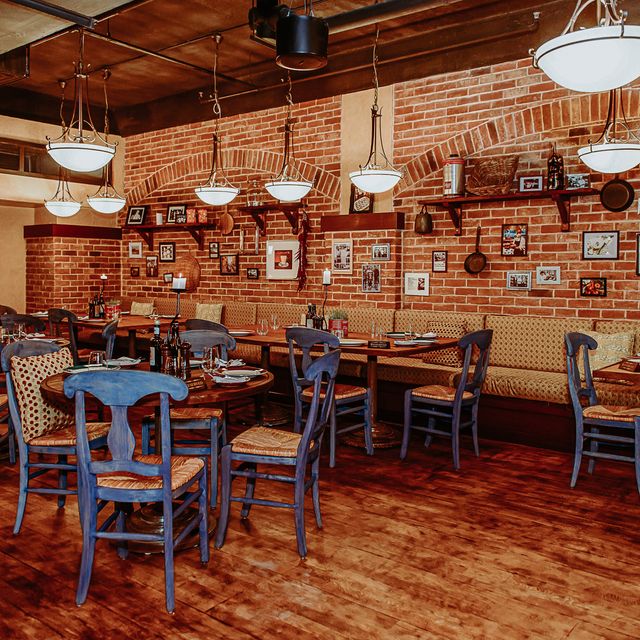The photograph depicts the interior of a charming, old-fashioned restaurant with a rustic yet cozy ambiance. The space features a warm, inviting setting with deep wooden floors and exposed red brick walls, which exhibit varying bricklaying styles, including straight and curved arrangements. Along the walls, diner-style booth seating is upholstered with vintage polka-dot patterned cushions, and some of the chairs, both wooden and metal with wicker seats, are adorned with cushions in diverse patterns.

The dining area includes an assortment of round and rectangular wooden tables, each set with plates, serviettes, and various condiments, arranged for a formal meal. Suspended from the wooden ceiling are numerous hanging bowl-like lamps that emit a soft, warm light, enhancing the overall ambiance.

The walls are decorative, adorned with a variety of objects such as old-fashioned photographs, antique cast iron frying pans, woven baskets, and other farm-like decorations, adding to the rustic charm. The shelves on the walls display more trinkets and cylinders of indeterminate use, contributing to the eclectic decor. Although the room is empty of people, the detailed setting and the lack of discernible text about its location suggest it's a cozy, well-decorated restaurant ready to welcome diners.